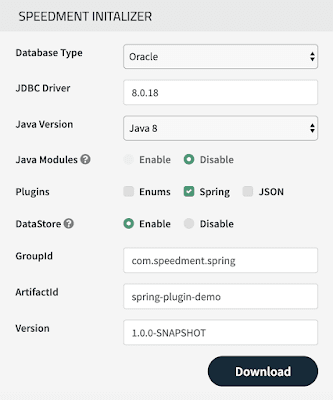The image features a screenshot of an online application interface, presented within a rectangular frame. The background color of the window is a soft off-white, providing a neutral backdrop for the content. The text within the window is displayed in black, ensuring clear readability. 

At the very top of the window, on a slightly darker gray bar, the title "Speed Mint Initializer" is prominently displayed. Below this title bar, the main section of the window is segmented into various interactive elements. On the right side of the window, there are several drop-down boxes labeled with corresponding titles, allowing users to make selections from predefined options.

Adjacent to these drop-down boxes, situated in the middle of the interface, are various radio buttons and checkboxes, offering additional user input choices and configurations. 

Moving to the left side of the window, in the upper left corner, there are a series of labels such as "Database Type," "JDBC Driver," "Java Version," "Java Modules," "Plugins," "Data Store," "Group ID," "Artifact ID," and "Version". These labels likely correspond with the drop-down boxes and other input fields scattered throughout the window, guiding users in specifying details pertinent to their task.

Finally, at the bottom right corner of the window, there is a prominent black "Download" button, positioned for easy accessibility once all the necessary information has been entered.